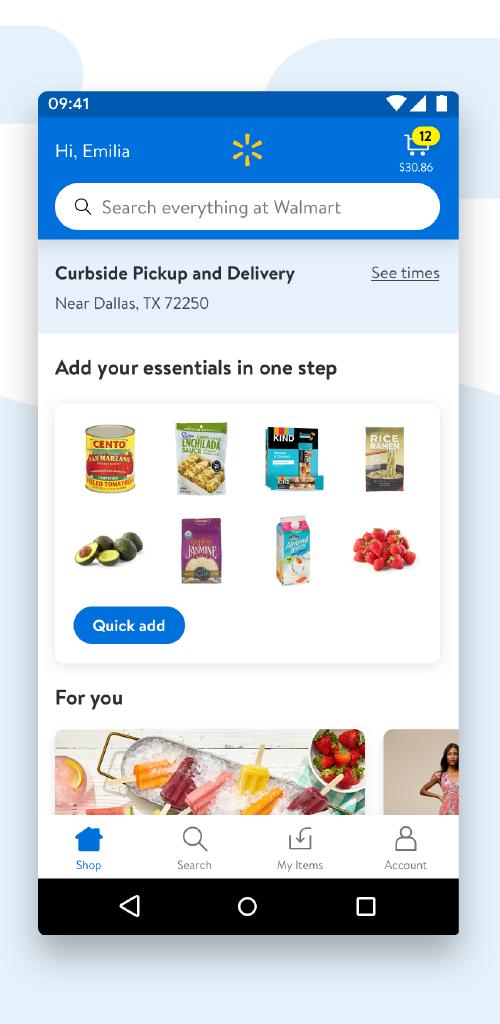The screenshot displays the homepage of the Walmart app on a smartphone. At the top, the app greets the user with "Hi, Amelia" next to the Walmart logo. There is a shopping cart icon in the upper right corner indicating there are 12 items in the cart totaling $30.86. Below, a prominent search bar is displayed with the text "Curbside pickup and delivery near Dallas, Texas, 72250." Beneath the search bar, the text "See times" is visible, followed by "Add your essentials in one step."

The screen features a selection of grocery items such as tomatoes and avocados under a section titled "For You." Toward the bottom, the basic navigation menu includes options labeled "Shop," "Search," and "My Walmart." At the very bottom of the screenshot, the Android navigation bar is also visible, featuring the standard back, home, and app switcher buttons.